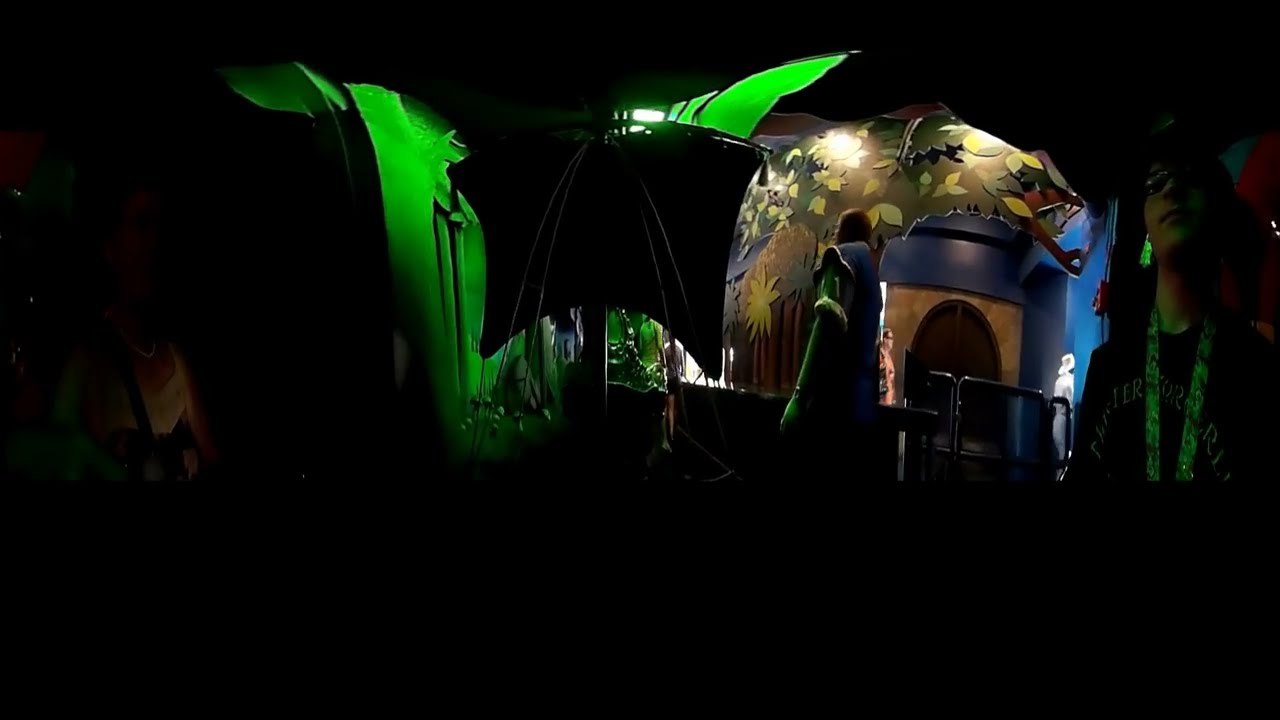This is a panorama of a very dark image featuring a central figure and a potential stage setting. On the right side of the image, there is a young person shown from the chest up, wearing glasses, a black t-shirt with indiscernible white letters, and a greenish-black lanyard around their neck. The background transitions into what appears to be a theater stage or a makeshift set with cut-out trees or palm trees and a dark brownish backdrop. There are some three-dimensional, fake leaves on the wall. Towards the middle part of the image, green light illuminates an area that resembles sails or a rectangular rounded shape. To the far left, parts of a playful mural in yellow and green, featuring flower shapes and bursts, are visible along with an archway and a fabric structure tinted green by the lighting. Thick black borders on the top and bottom frame the image, constricting the view and adding to the overall darkness, suggesting that the photo might have been taken as a panoramic selfie at a stage or creative exhibit.